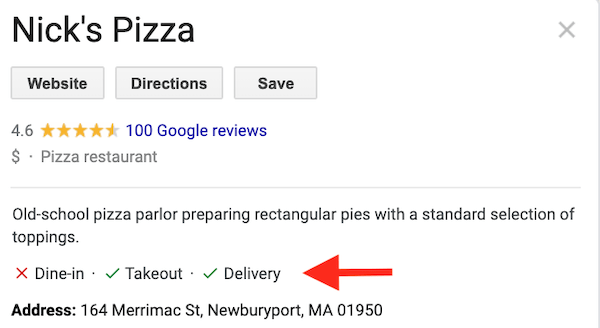The image depicts a Google search result for a restaurant named "Nick's Pizza." At the top of the search result, the restaurant's name, "Nick's Pizza," is prominently displayed. Directly below the name, there are three interactive buttons labeled "Website," "Directions," and "Save." Further down, the restaurant's rating of 4.6 stars is shown, accompanied by the note "100 Google reviews."

In terms of pricing, the restaurant is marked with a single dollar sign, indicating a relatively inexpensive option. It is categorized under "Pizza restaurant." Below these details, a brief description of Nick's Pizza is provided: "Old-school pizza parlor preparing rectangular pies with a standard selection of toppings."

Additionally, an arrow points to the word "Delivery," suggesting delivery options are available for this establishment.